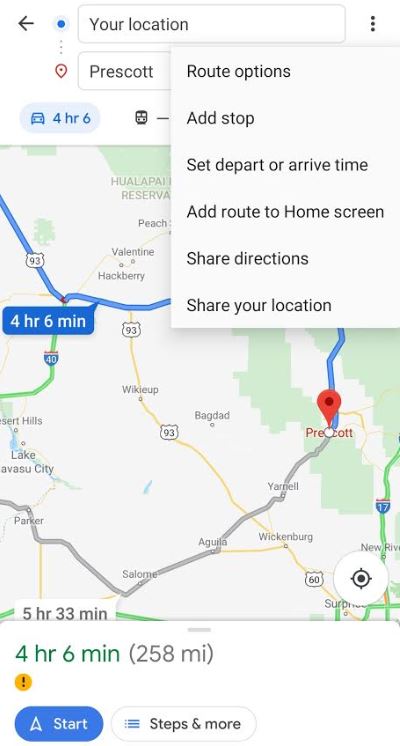This image, captured from a cell phone screen, showcases a navigation map application. The background is a detailed map, with a white rectangular overlay at the forefront displaying six interactive options. At the top of the overlay, in bold black text, is the heading "Route options." Beneath this, several functions are listed: "Add stop," "Set depart or arrive time," "Add route to home screen," "Share directions," and "Share your location."

Above the overlay, a blue dot represents the user's current location, labeled "Your location." The destination, "Prescott," is marked with a pin. To the side of these markers, an icon of a car is displayed alongside the estimated travel time of "4 hours 6 minutes."

At the bottom of the screen, a driving route is depicted, instructing the user to travel down Highway 93 before curving towards Prescott. This route is marked with a red pin at the destination and indicates that the journey will take approximately four hours and six minutes. Additional options such as "Start" and "Steps & more" are visible for further navigation details.